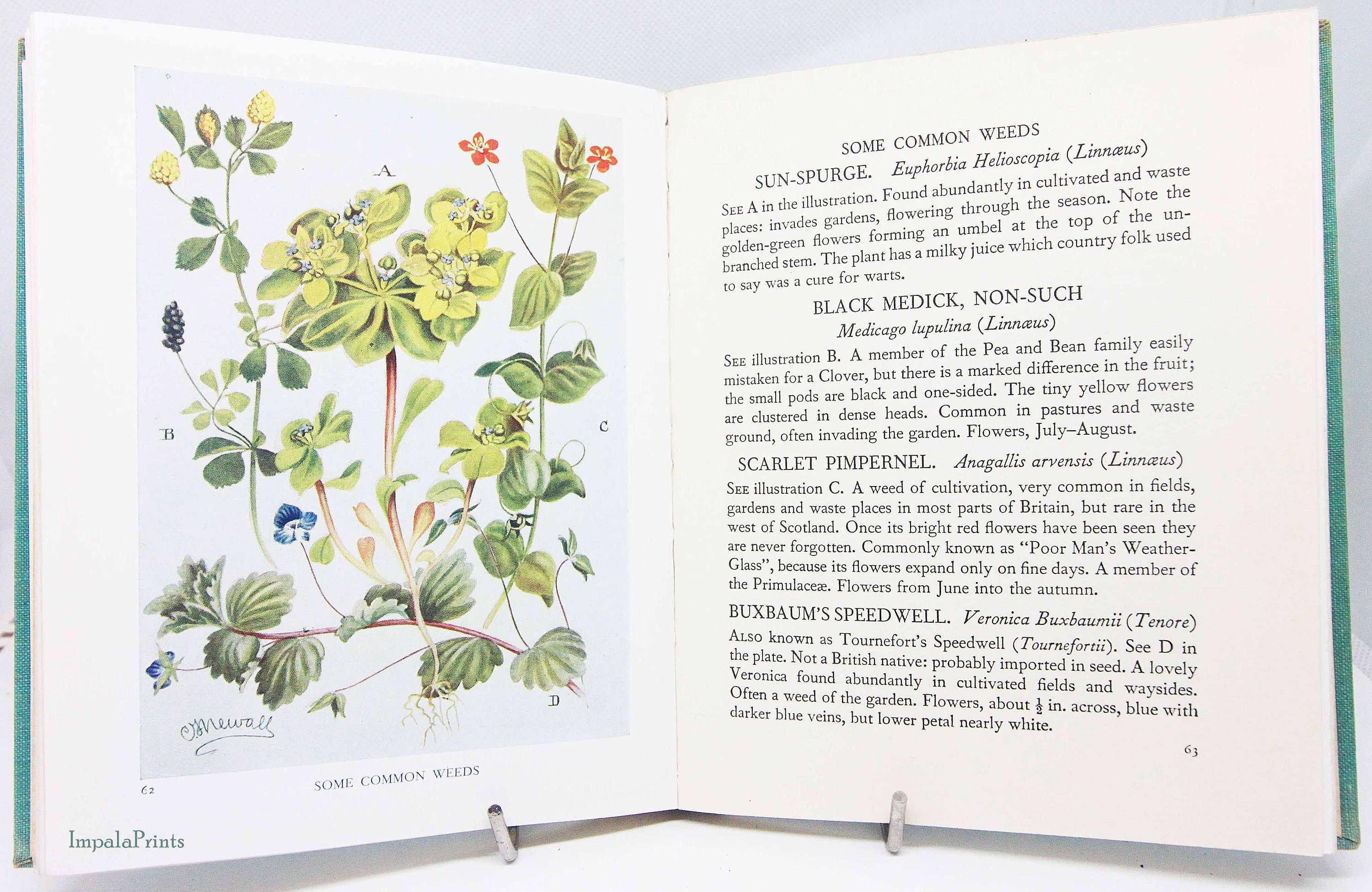An open book rests on a wire book holder, typically used for cookbooks. The holder, which is gray or grayish-white, is partially visible, primarily showing the front section that supports the book. The book has a greenish cover, with just the edge peeking out. It is open to page 63, revealing a detailed section titled "Some Common Weeds." The right-hand page lists various plants such as sun spurge, black medic, and scarlet pimpernel, accompanied by their Latin names and descriptions. The left-hand page features intricate illustrations of these plants, depicted in vibrant red, yellow, and other colors, likely representing different wildflowers that correspond to the descriptions on the right.